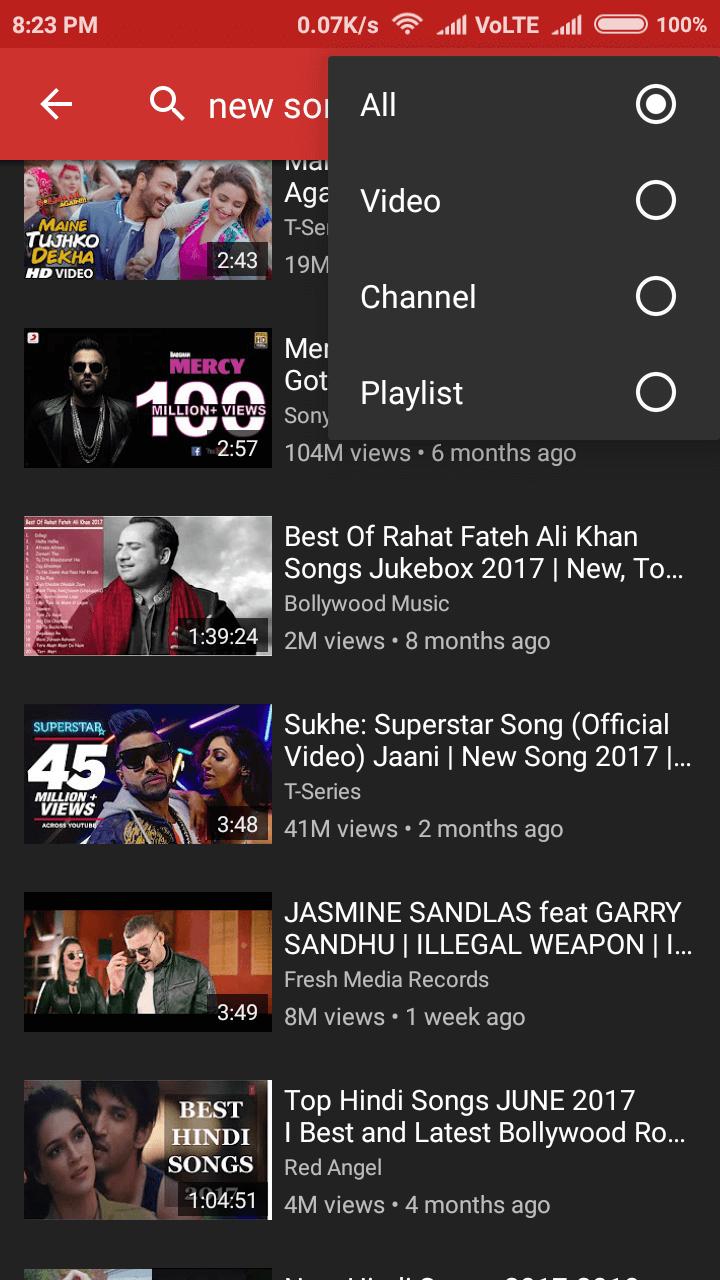This is a screenshot of a mobile phone displaying a music application. 

At the very top of the screen, there's a red status bar with white text displaying the time "8:23 PM," the data transfer rate "0.07 KB/s," along with full WiFi and mobile signal bars. The indicators show "V-O-L-T-E" and the battery is fully charged at 100%.

Below the status bar, there is a red navigation bar featuring a white magnifying glass icon and the text "New Songs" in white font. Immediately beneath it, a grey pop-up menu is visible with "All" selected in white font. This menu contains additional options labeled "Video," "Channel," and "Playlist."

The main content area shows the results of a search for new songs, displayed as six YouTube video thumbnails in a grid format. The top portion of the screen is partially obscured by the pop-up menu, covering the titles of the first two video thumbnails. The visible thumbnails suggest that the videos are related to Indian music, specifically Bollywood. Some of the video titles are legible, such as "Best of Rahat Fateh Ali Khan Songs Jukebox 2017."

Overall, the image showcases a search for new songs on a music app, emphasizing Indian and Bollywood-themed content.